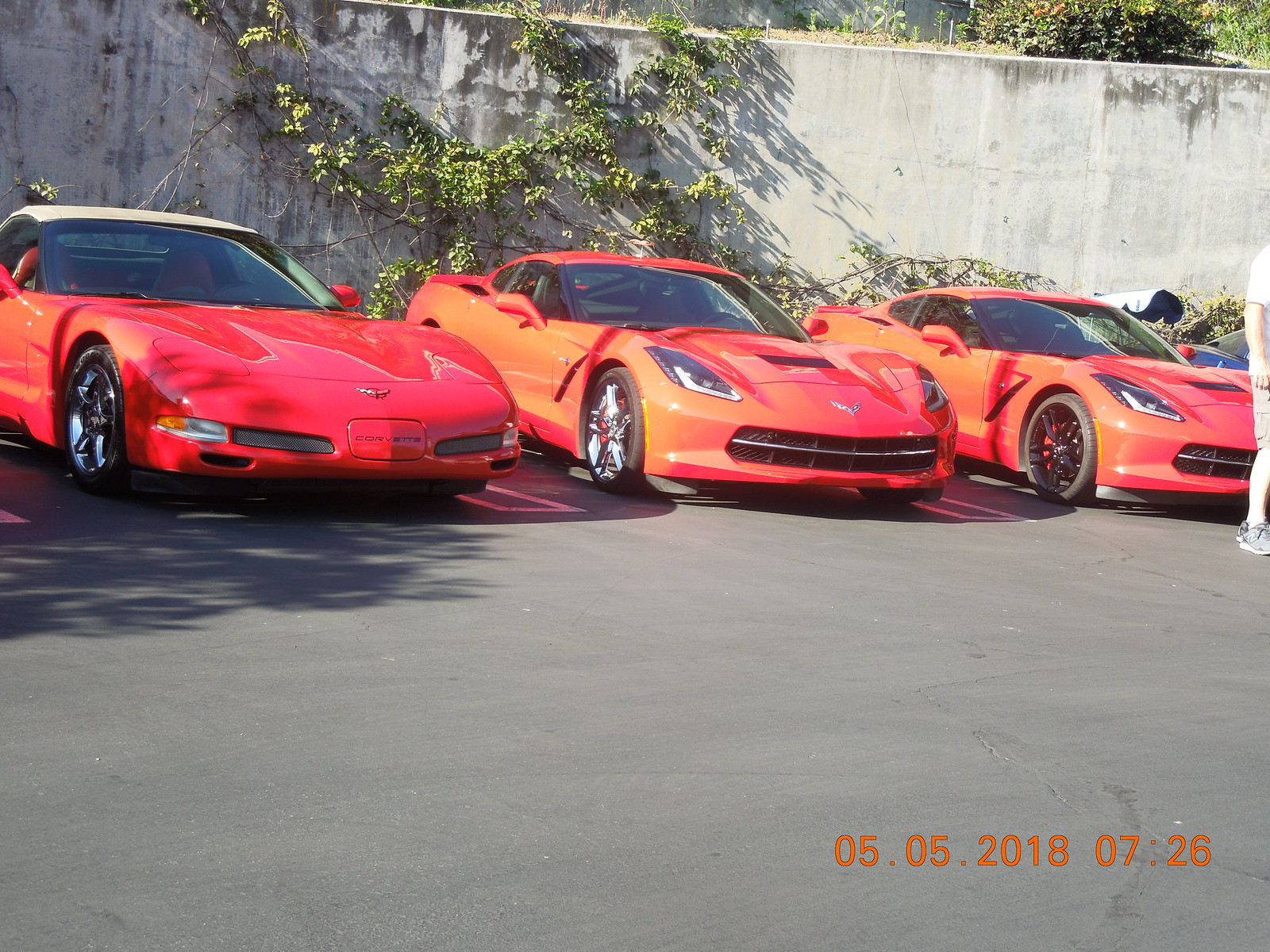The photo features three clean and shiny red Corvettes parked in a parallel formation on a grayish concrete pavement, clearly indicating they are luxury sports cars. Notably, one Corvette appears to be an older model, while the other two are much newer. In the background, the cars are positioned against a grey concrete wall adorned with green vegetation trailing down from the top. A blue car is barely visible next to one of the Corvettes. The bottom right corner of the image contains an orange timestamp reading 05.05.2018, 07:26. Additionally, a partial view of a person can be seen, with a visible leg and arm clad in shorts and grey sneakers. The Corvettes’ shiny hubcaps catch the light, although one car has a distinctive black hubcap. Interestingly, two of the cars have their headlights illuminated.